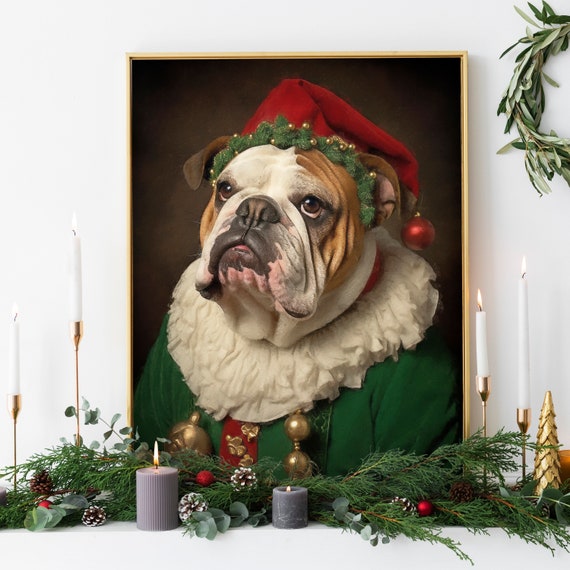A humorous and detailed painting depicts a French Bulldog (or possibly a Boston Bulldog) dressed in an elaborate, historical Elizabethan outfit, featuring a white frilled ruffle collar and a green tunic. The dog, with its droopy mouth, brown and white face, soft brown eyes, slightly pushed in snout, and heavy jowls, faces slightly to the left while turning its head towards the viewer. The Bulldog wears a red stocking cap adorned with green pine branches and small gold ornaments, with a red Christmas ball hanging from the tip. This Renaissance-style portrait, with a dark blurred brown background, is set in a narrow gold frame, leaning against a white wall. The frame is perched on a white shelf decorated for Christmas with green pine branches, snow-tipped pine cones, red Christmas balls, and gray pillar candles, contributing to a festive atmosphere. On either side of the frame are tall, lit taper candles in gold holders. In the upper right corner of the photograph, part of a simple winter greenery wreath is visible on the wall.